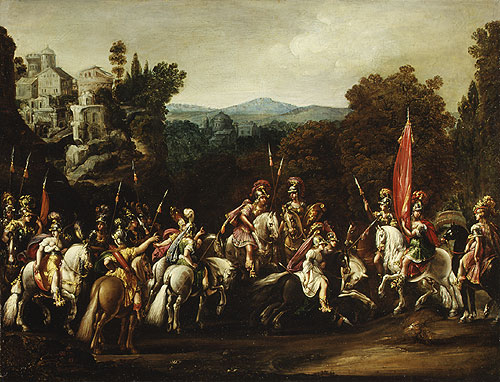In this detailed and evocative painting, a group of medieval soldiers, likely reminiscent of Roman or ancient Greek warriors, are mounted on their horses, poised in front of an imposing castle and a richly varied landscape. The soldiers, dressed in ornate armor and helmets adorned with red feathered crests, wield spears and one proudly holds aloft a red flag. One striking horse on the right with a long, flowing white mane stands with one foot raised, adding a dynamic element to the scene.

The castle in the background features several round, spiraled towers and is built into the side of a mountain. To its left, the edge of the mountain peaks through, while to its right, a dense green tree and another more brownish tree stand tall. Beyond the immediate foreground, rolling hills and mountains stretch across the horizon, fading into a distant blue and amber tint, their thick foliage rendering them almost impenetrable to the eye. The sky above is tumultuous, filled with dark gray and white clouds that cast a somber mood over the tableau. The overall scene is a vivid and dramatic portrayal of an ancient, battle-ready force set against a richly detailed and textured environment.